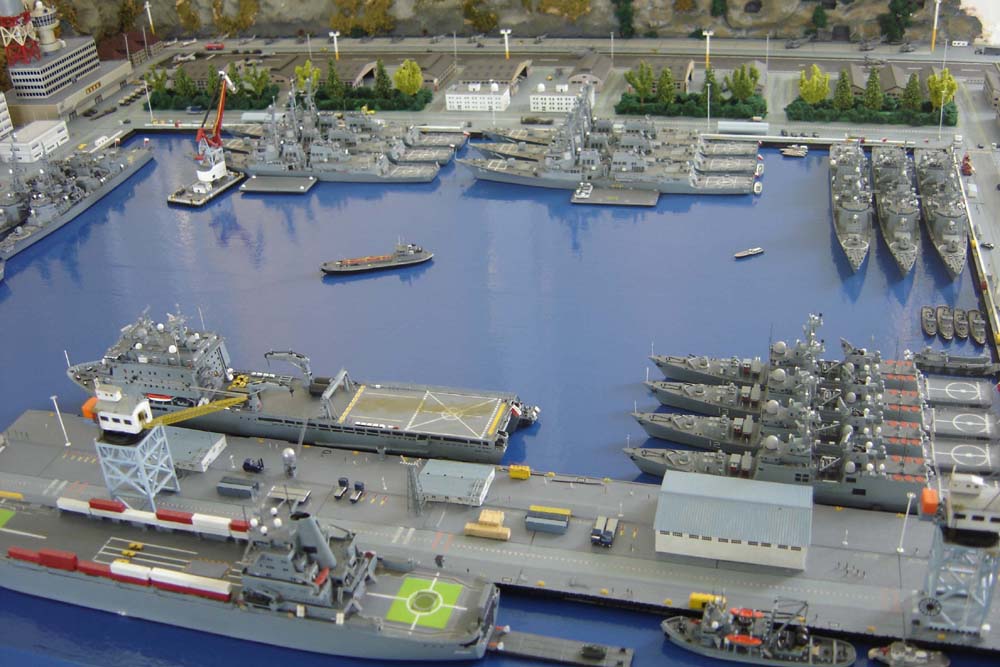This photograph showcases a detailed miniature model of a naval shipyard. The scene features a variety of meticulously crafted military ships lined up in a harbor with flat, dark blue water. Prominently, the model includes a large aircraft carrier alongside several destroyers, battleships, and cruisers, the latter of which have helipads on their sterns. Gray is the predominant color for all the ships. Notable elements within the model include dome-shaped bunkers, various hangars with gray roofs and white walls, and a towering cylindrical structure adorned with red and white scaffolding. We can also observe intricate details such as miniature trees, bushes, parked model cars, and busy roads running through the shipyard. Additionally, there's a small white crane with a red arm situated near one set of cruisers and a moving boat in the water that emphasizes the realism of the scene. This highly detailed and realistic depiction captures the bustling activity and infrastructure of a naval shipyard in miniature form.